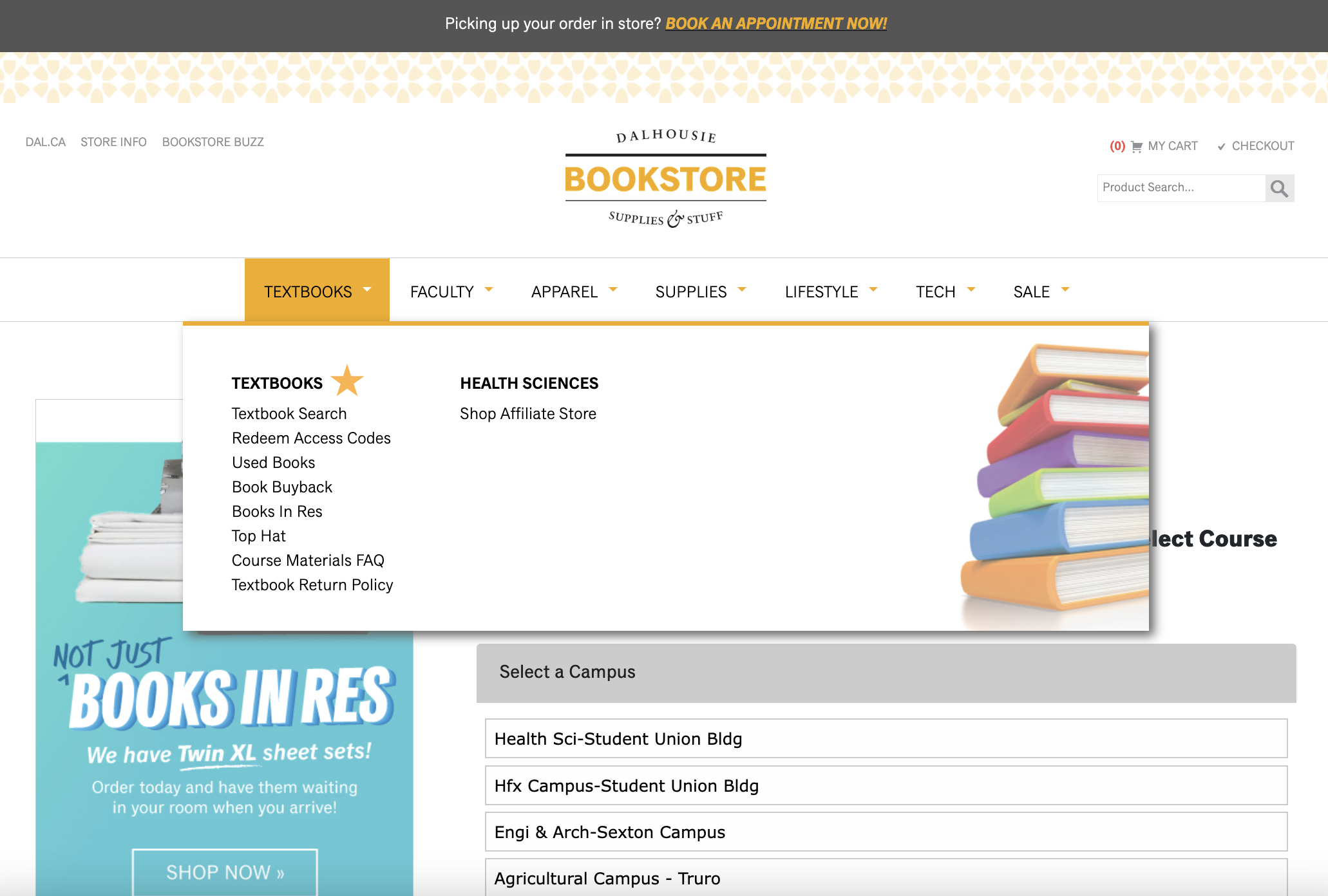The image is a screenshot of a bookstore's website. At the top, a gray banner spans across with text that reads, "Picking up your order in store? Book an appointment now." Below this banner, prominently located in the center, is the bookstore's logo which reads "Dow Dowsy Bookstore."

On the left side, there is a navigation menu featuring options such as "Store Info," "Bookstore Buzz," and what looks like "DLC." On the far right, there are icons for "My Cart" and "Checkout," followed by a search field with a magnifying glass icon.

Directly beneath the logo, another menu lists various categories. The current highlighted option is "Textbooks," shown in gold, with other categories like "Faculty," "Apparel," "Supplies," "Lifestyle," "Tech," and "Sale" remaining in white. Under the "Textbooks" tab, a submenu appears, displaying bold black text such as "Textbooks," "Health Sciences," and "NBC Shop Affiliate Store."

The main content of the page features an assortment of books stacked together, creating a visually busy background. To the side, there are additional site options for selecting different campus locations, including the "Campus Health Science," "Student Union Building," and "Agricultural Campus," totaling five possible selections.

On the left side of the page, a small box adver­tises, "Not just books! In res: We have Excel sheet sets," with a prompt to "Shop Now."